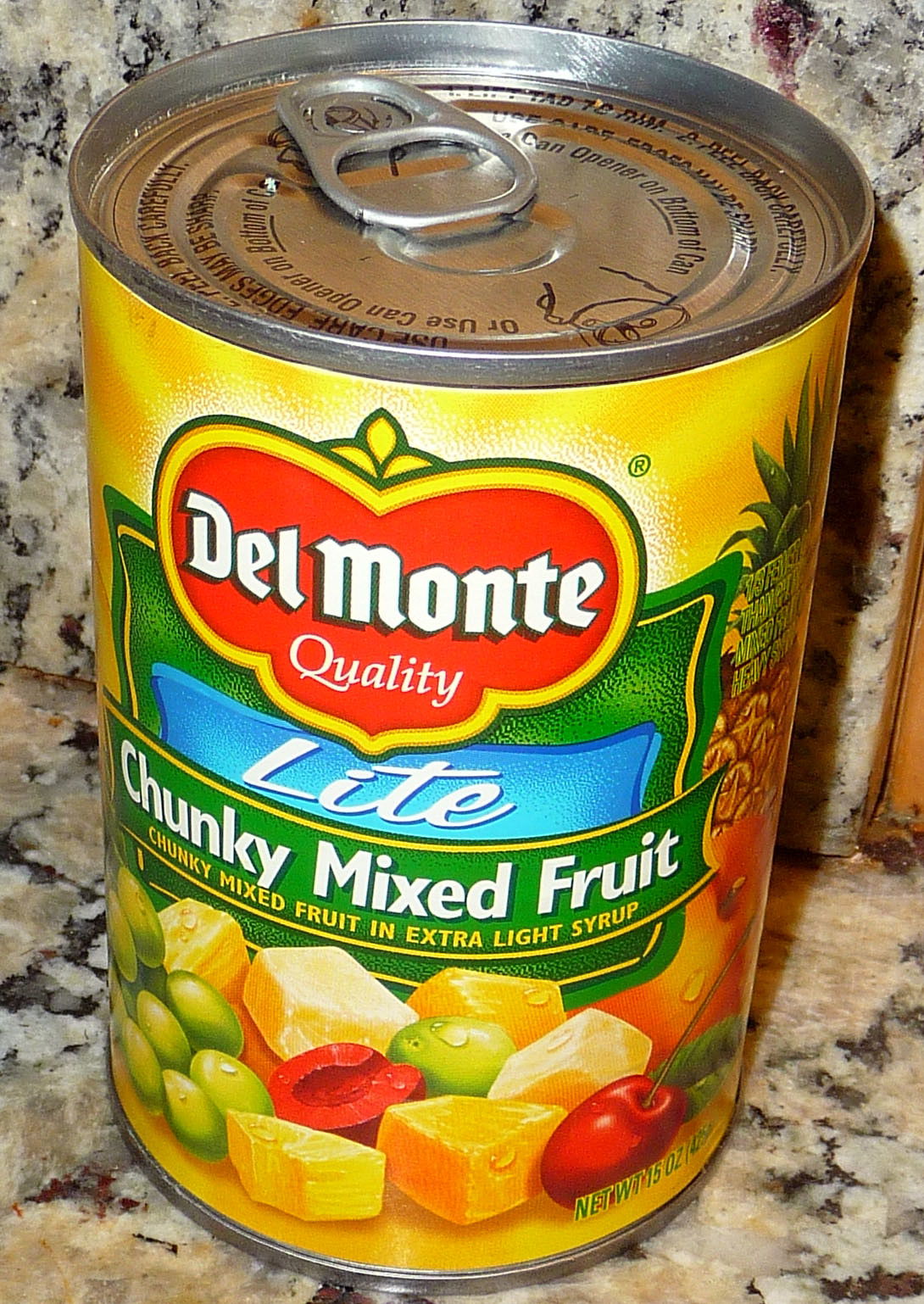This is a vertically oriented photograph of a Del Monte Chunky Mixed Fruit can, captured from a slightly elevated, left-leaning downward angle that introduces a touch of foreshortening. The can is positioned on a marble surface, with a splash guard suggesting the edge of a kitchen countertop against the wall.

The can features a metal top equipped with a pull-tab, reminiscent of a soda can. The label is predominantly yellow, showcasing a prominent red Del Monte quality logo outlined in yellow at the center. Below the logo, there is a smaller, white "Light" text within a blue rectangle, followed by the bold, white text "Chunky Mixed Fruit." Continued in yellow font is the descriptor "Chunky Mixed Fruit in Extra Light Syrup," indicating the contents and their preparation.

The lower part of the label is adorned with vibrant illustrations of various fruit pieces, representative of the can’s contents.